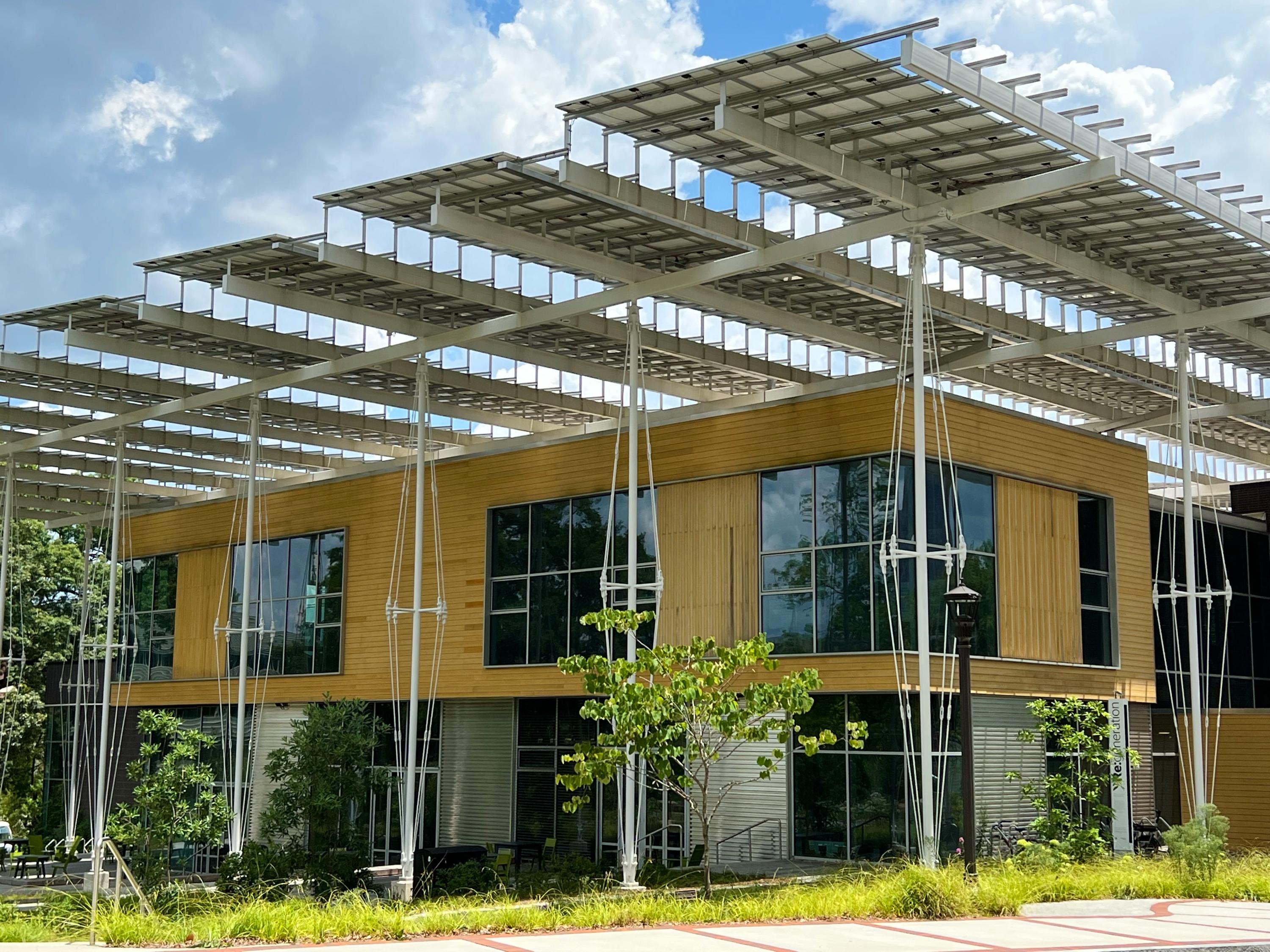This close-up photograph captures the lower half of a futuristic, two-story building, possibly a house. The design features an elaborate structure with six metal beams supporting a large array of solar panels mounted on the roof. The bottom floor is adorned with metal slats and floor-to-ceiling windows, while the second story showcases a tan or wooden exterior surrounding three massive windows. Fancy-looking beams, which taper and flare out, add to the modern aesthetic. The building is surrounded by light landscaping, including grass, small trees, and a black pole light. There also appears to be gray stairs on the left side, enhancing the overall intricate design of this eco-friendly, solar-paneled building.